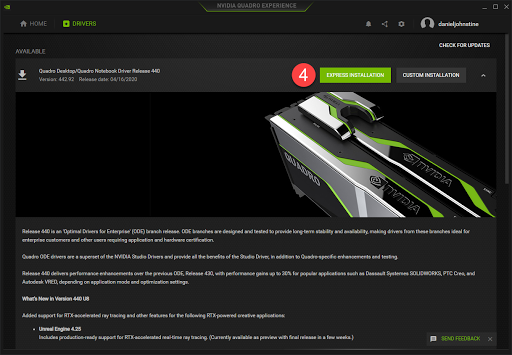This is a detailed and cleaned-up caption for the image described:

---

This image is a screenshot from the "NVIDIA Quadro Pro Experience" website. The site’s name is prominently displayed in an inverted tab at the top center of the page. Below this header, a black menu bar is present, with the "Home" and "Drivers" options on the left side; the "Drivers" tab is highlighted in green. 

Underneath the menu bar, there is a designated box titled "Quadro Desktop/Quadro Notebook Driver Release 410." On the same row to the right, there are two installation buttons: a green "Express Installation" button and a gray "Custom Installation" button. Adjacent to these buttons is a red circle with the number "4" inside it.

Accompanying the installation options is a product photograph depicting what appears to be a type of processor or computer accessory. The product features a sleek, silver casing accented with green highlights and black sections, set against a black background. Below this image, there is a block of white text spanning six or seven lines, although the text is too small to read clearly, even when zoomed in. 

At the bottom of the screenshot, a bullet-point section is visible, likely labeled "What's New in Version 4.40." 

In the upper right corner of the screen, a user's avatar—depicted as a silhouette—accompanies the username "Daniel Jonathan". Additionally, the browser window controls, including the "X" (close), "minimize," and "maximize" buttons, are located at the top right.